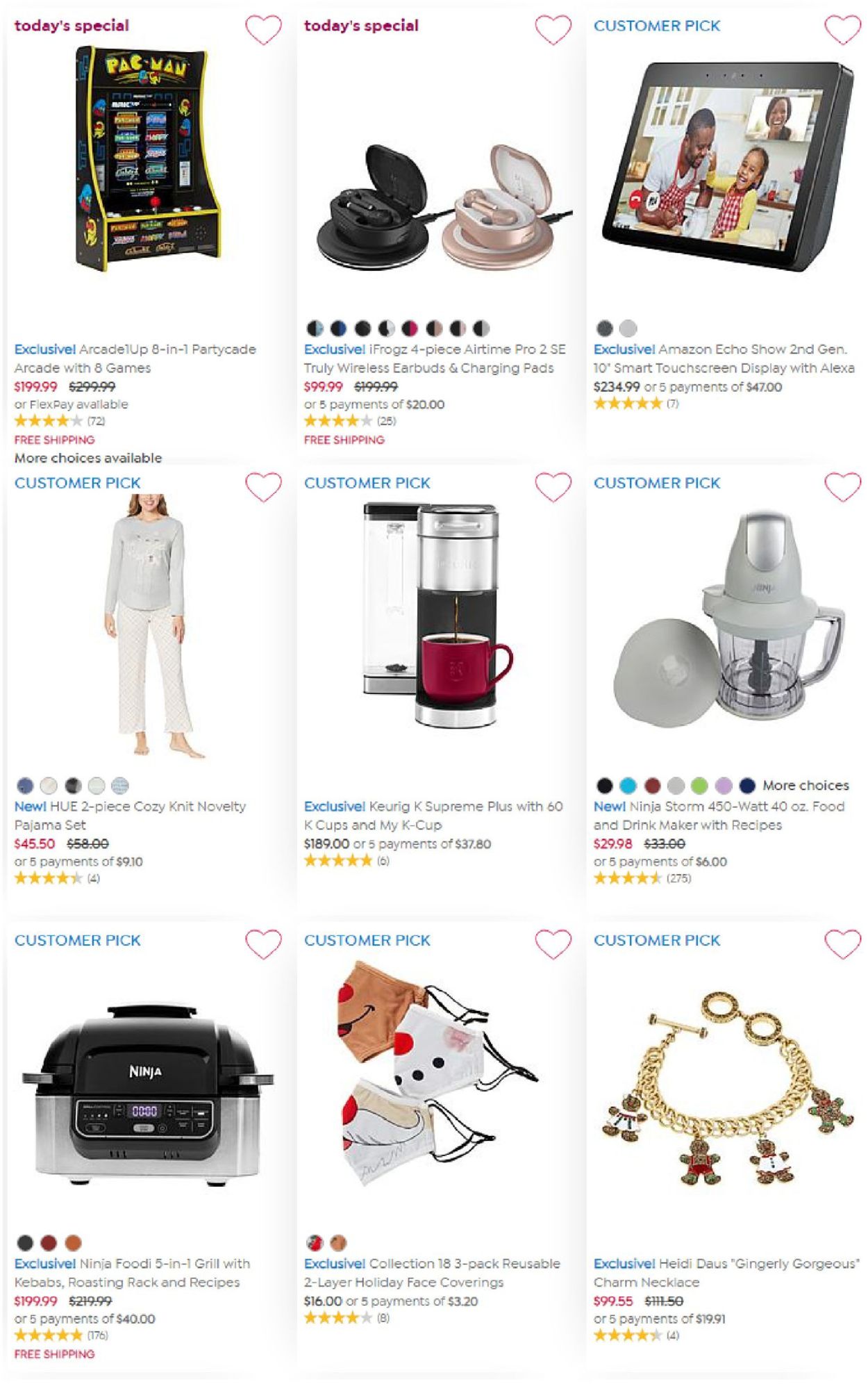Here's a meticulously detailed caption for the described image:

---

A screen capture from a retail website showcasing various items for sale is organized into three rows of three images, totaling nine items. 

1. The first item, marked as "Today's Special" in purple accompanied by a small purple heart, is a Pac-Man arcade machine labeled as "Exclusive" in blue. There is some ambiguity in the text which could read "5-in-1" or "8-in-1" arcade game system, with price and star rating details visible.

2. The second item, also under "Today's Special" with a purple heart, features wireless earbuds. The display shows two color options - black and rose gold. The price is highlighted in red along with overlaid star ratings.

3. The third item is an Amazon Echo tablet, marked as "Customer Pick" in blue along with a purple heart. The tablet is black, and the image depicts a family using it in a kitchen setting. Pricing and rating details are present.

4. The fourth item portrays a woman wearing gray and white pajamas. Multiple color selections are indicated by various color icons. Price and customer ratings are included.

5. The fifth item is a silver and black coffee machine, designed to use K-cups. This product is a "Customer Pick" marked in blue with a heart icon, depicted with a red coffee cup. The price and reviews can be seen.

6. The sixth item appears to be a kitchen appliance in gray. While the specifics of the item are unclear due to hard-to-read font, it features several color options: black, teal, burgundy, gray, orange, green, lavender, and navy. Pricing and ratings are shown.

7. The seventh item is an air fryer in black and silver with a digital display. The product includes visible price and customer reviews.

8. The eighth item shows an assortment of Christmas-themed face masks. One is designed like Rudolph in red and brown, another as a snowman in white with a coal mouth, and a third as Santa with a white beard. Prices and ratings accompany the display.

9. The final item is a gold bracelet adorned with gingerbread man family charms. The bracelet’s price and customer reviews are provided.

---

This detailed caption captures the specifics of each item and its presentation on the website, providing a comprehensive overview of the displayed products.